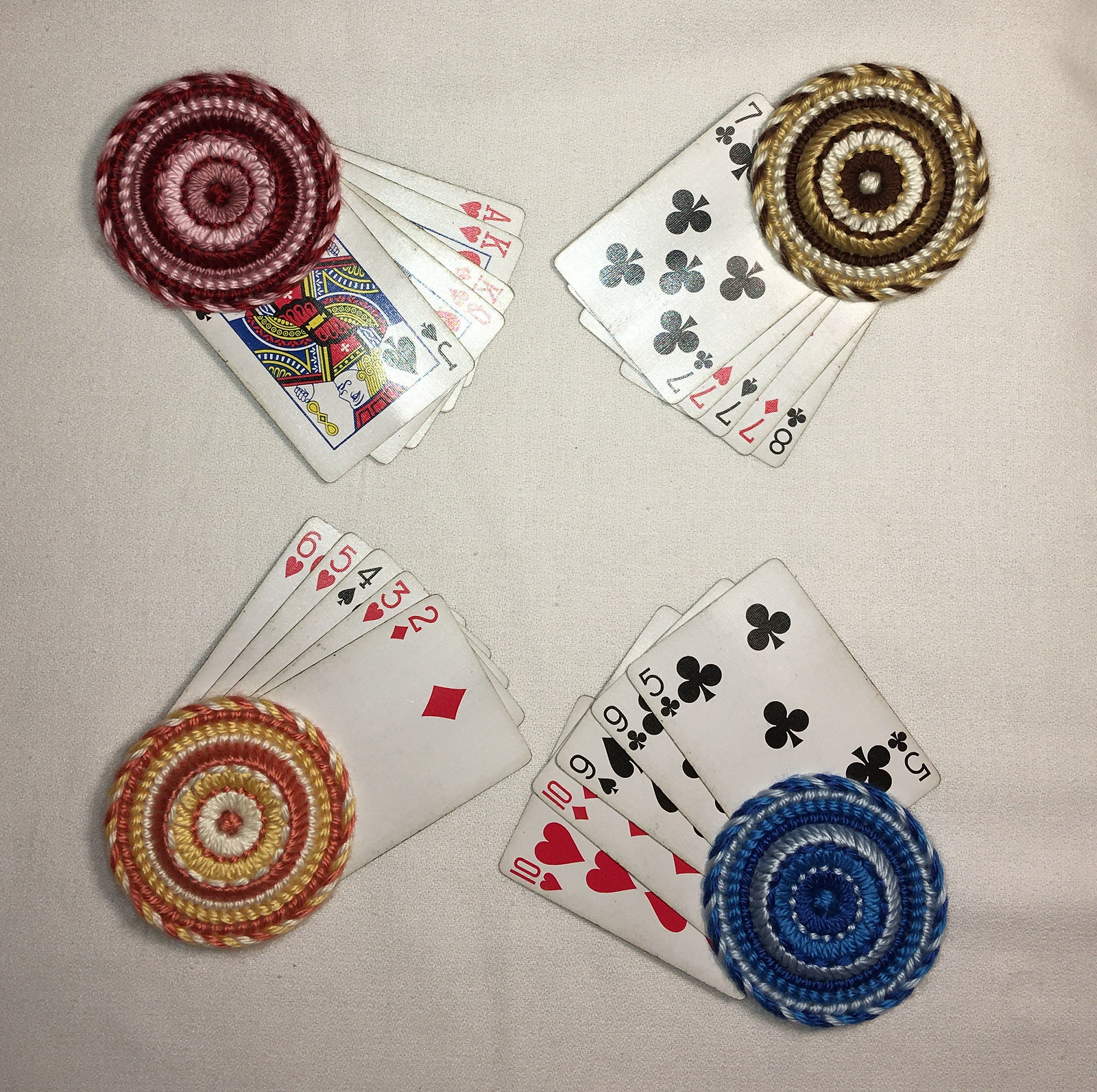This top-down photograph captures an arrangement on an off-white or creamy white tablecloth. At each corner of the image is a distinct hand-knit coaster, each large enough to hold the base of a typical drinking glass. The coasters each boast unique color schemes: the top left coaster features varying shades of red; the top right exhibits different shades of white and brown, reminiscent of 1970s aesthetics; the bottom left coaster is adorned with shades of orange and yellow; and the bottom right showcases medium and light blues.

Underneath each coaster lies a set of playing cards, each combination meticulously facing up. The set beneath the top left coaster displays a jack, queen, king, king, and ace. The cards under the top right coaster reveal four sevens and an eight. The lower left ensemble consists of a six, five, four, three, and two. Lastly, under the bottom right coaster, there are two tens, two nines, and one five. Based on the given hands, the top left combination appears to be the strongest, suggesting a winning poker hand, although the exact poker rules might influence this outcome.

The photograph effectively captures a moment filled with rich textures and colors, intertwined with elements of leisure and nostalgia.